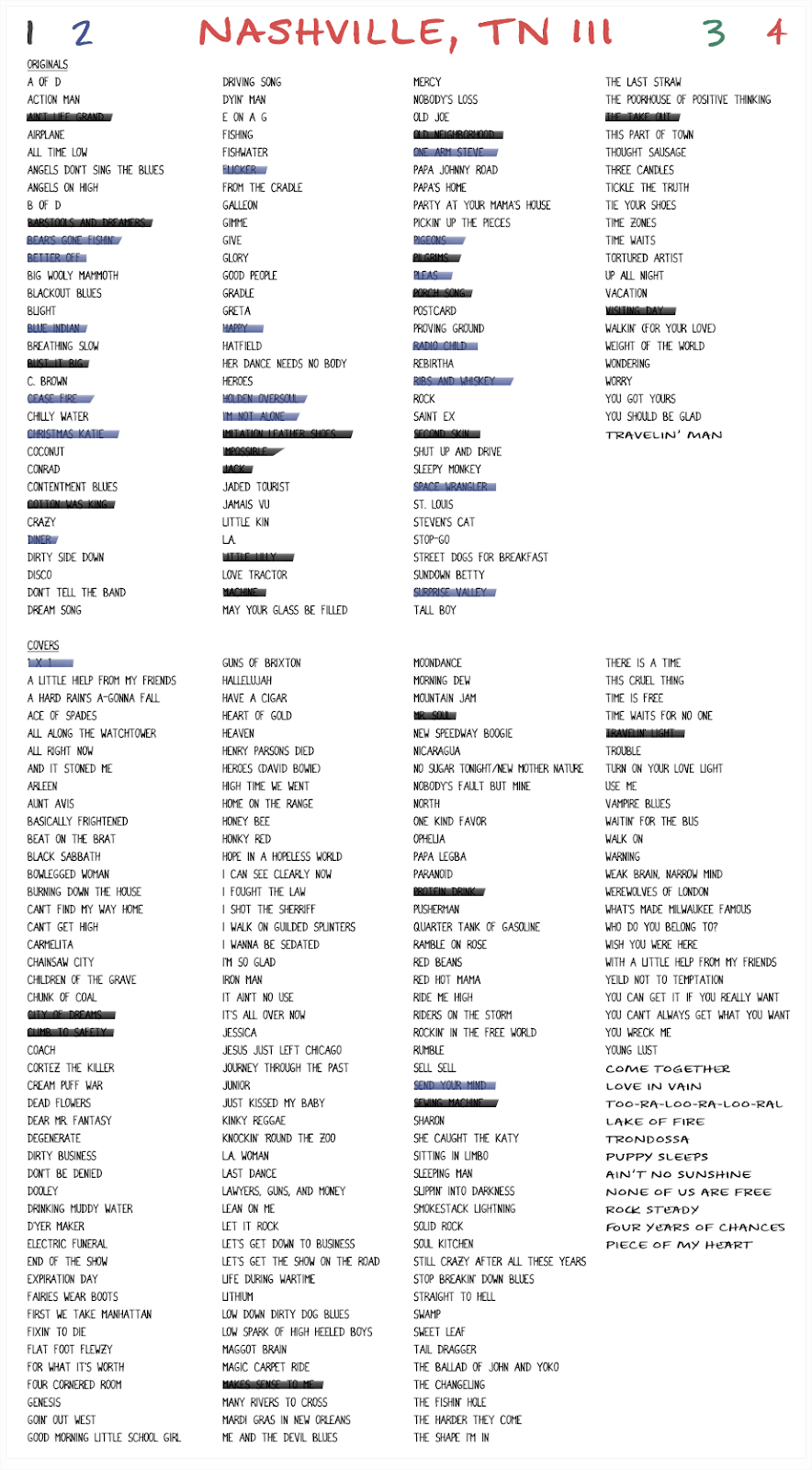The image is a vertically-oriented artwork featuring four columns of text at both the top and bottom. At the top of the image, in thin, cartoon-style writing, it reads "Nashville T.N." with three lines drawn beside the text. The top corners of the image contain the numbers 1, 2, 3, and 4; specifically, 1 and 2 are in the left corner, and 3 and 4 are in the right corner. These numbers categorize lists of song titles.

In the top left corner, under the heading "Originals," there are several song titles listed:
1. A of D
2. Action Man
3. Airplane
4. All the Low
5. Angels Don't Sing the Blues

Some of these titles are crossed out, with some lines drawn in black and others in blue.

The adjacent column continues with more song titles:
1. Driving Song
2. Dying Man
3. E on A
4. G
5. Fishing
6. Fish Water

The top right section of the image has two more columns of song titles. The third column includes:
1. Mercy
2. Nobody's Loss
3. Old Joe

The fourth column lists:
1. The Last Straw
2. The Poor House of Positive Thinking
3. This Part of Town
4. Thought Sausage

These columns are presented on a plain white background, creating a clear and straightforward layout for the viewer to follow.